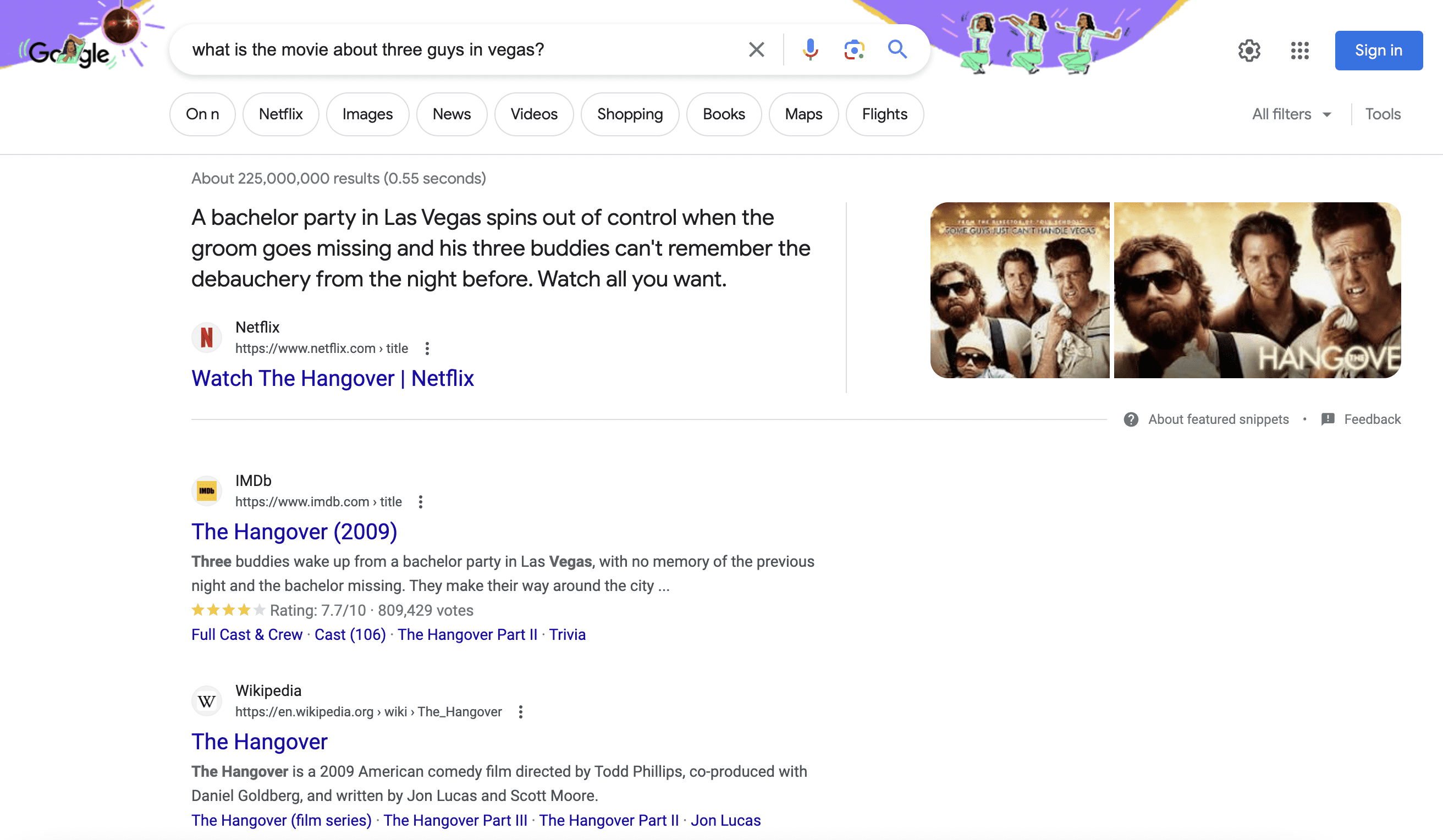The image depicts a detailed screenshot of a Google search page, specifically searching for information about the movie "The Hangover." The background is predominantly white, featuring Google's signature layout. At the top, there's a unique Google Doodle showcasing some purple hues and people dancing, indicating a special celebration or event. 

The main search query in the search bar reads, "what is the movie about three guys in Vegas?" Below the search bar, several suggested searches are listed. The primary search result outlines, "A bachelor party in Las Vegas spins out of control when the groom goes missing as three buddies can't remember the debauchery from the night before," followed by a direct link to watch the movie on Netflix.

To the right, there are two thumbnail images from the first "The Hangover" movie. Above these thumbnails, there are typical Google account management options, such as the sign-in button, settings cog, and additional filters/tools buttons.

Following the Netflix result, the next major result comes from IMDb, providing information about the 2009 release of "The Hangover," including cast and crew details, trivia, and a nod to "The Hangover Part II." Below the IMDb result, there is a link to the Wikipedia page for "The Hangover," offering more detailed and unbiased information about the movie, its sequels, and the director, Jon Lucas.

Overall, the image encapsulates the entire search experience for someone looking up information about "The Hangover," highlighting key sources like Netflix, IMDb, and Wikipedia, along with visual content and standard Google functionality.